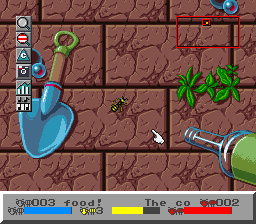This image is a screenshot from a cartoonish video game, featuring vibrant and playful graphics akin to a children's cartoon. At the center, there's a brick wall dotted with various interactive elements. Among these elements is a hand shovel and a glass bottle, which together suggest a game objective. Leaves are seen protruding from the wall, adding a natural touch to the scene. A bee hovers near the wall, marked by a pointing finger indicating a possible task, perhaps to trap the bee inside the glass bottle. Above, there's a mysterious circular globe resembling a marble, accompanied by a red rectangle with a smaller square inside it, suggesting a highlighted area or important icon, though its purpose is unclear due to its small size.

At the bottom of the screenshot, the game's interface displays important player statistics. The text reads "003 food!" indicating a food count. There are three colored meters: a full blue meter with a blue ant icon in front, a yellow meter slightly over halfway full with a yellow ant icon, and a fully filled red meter with a red ant icon. These meters likely represent different resources or stats necessary for gameplay.